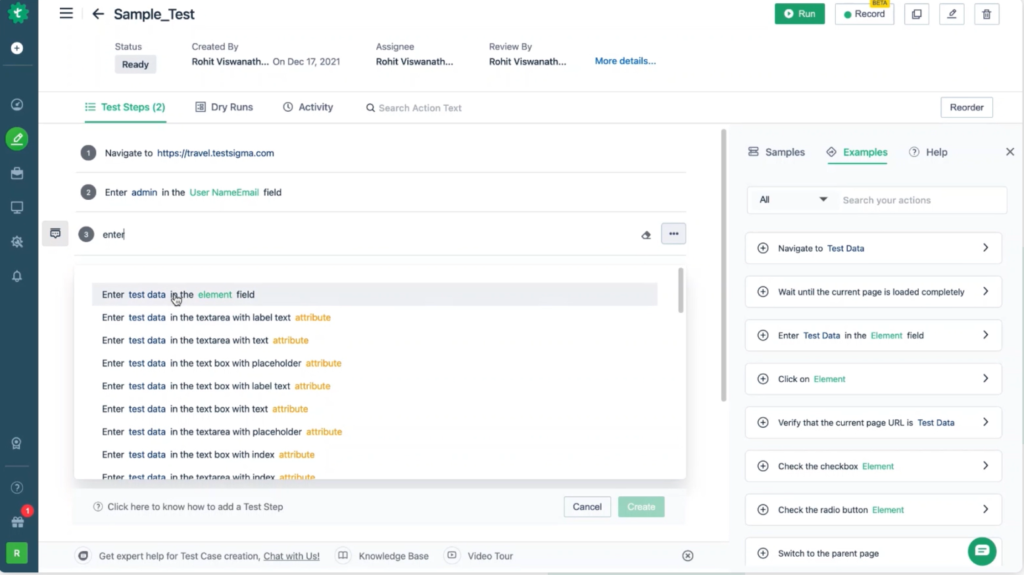This image is a screenshot of an administrative software page with a white background. On the left side, there is a narrow, dark blue sidebar menu featuring several icons. At the very top of this sidebar, there is a green circle, followed by a small white circle with a black plus sign, likely used to expand the sidebar. Below that, another larger green circle with a white emblem is visible. Further down, there is a small bell icon for notifications, and at the very bottom, there is a green square accompanied by a gray icon above it and a red circle with the number "1" inside it, indicating a notification or alert.

On the main page, at the top left corner, "sample_test" is written in dark gray font. Below this, a menu with categories such as "Status," "Created By," "Assignee," and "Reviewed By" is displayed. Further down, another category section lists "Test Steps," "Dry Runs," "Activity," "Search," "Action," and "Test."

Within this section, detailed instructions are provided, though some text is too small to read. It includes steps like "Navigate to [web address]" and "Enter admin in the [field]." There are dropdown menus and repeated prompts to "Enter text data in the [field]."

On the right side of the main content area, there is an additional sidebar titled "Samples, Examples, and Help," containing a long list of items that further aid navigation and functionality within the software.